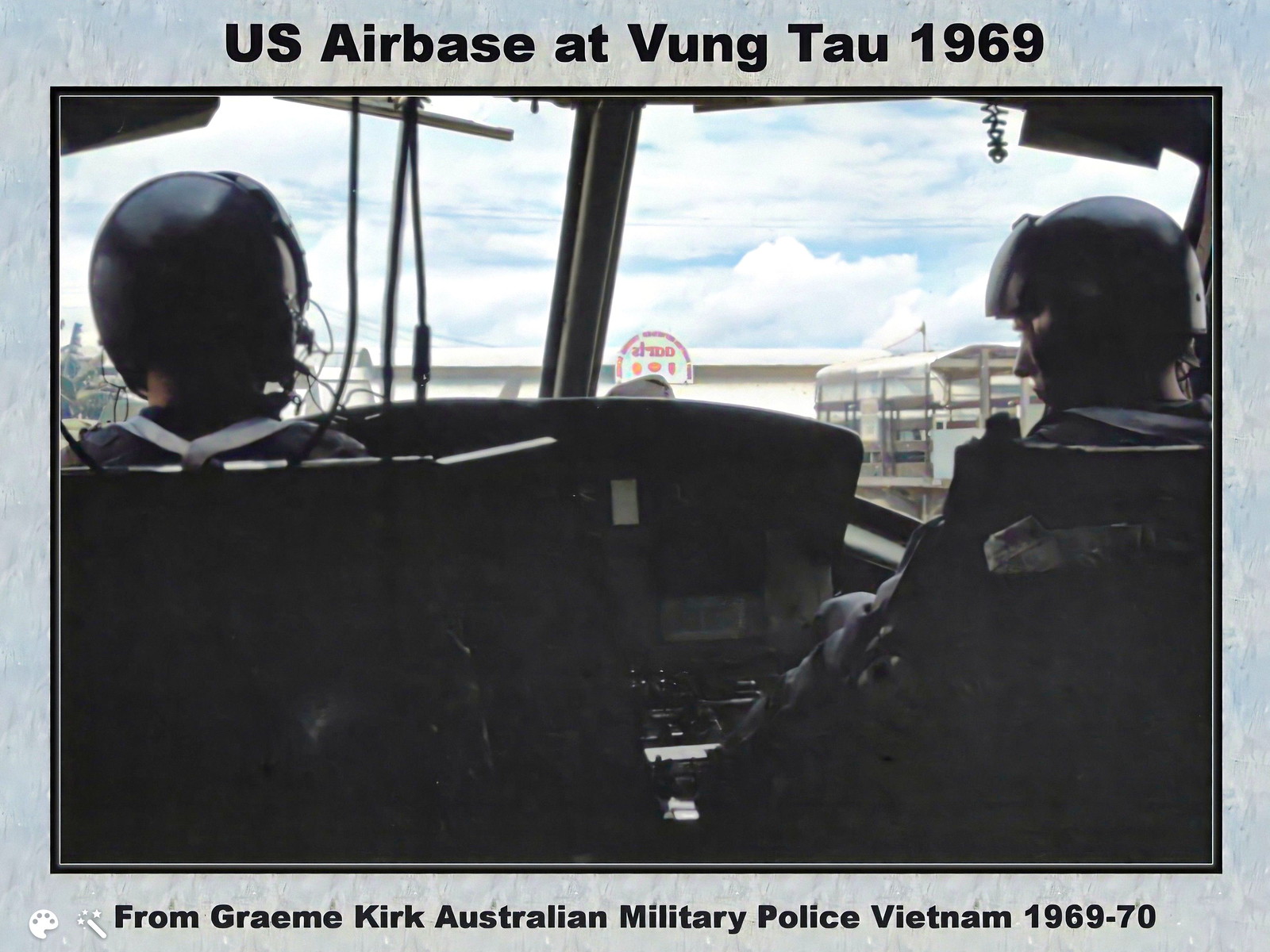A historical photograph from the U.S. Air Base at Vung Tau, dated 1969, captures two men seated in an airplane. Both individuals are equipped with helmets, and the man on the left is wearing a headset, possibly receiving or transmitting communication. The vantage point of the photograph is from the rear, as if the person taking the picture is seated directly behind them. The scene suggests that the aircraft is stationary, not yet airborne. Notably, the photo includes captions and details, indicating it's from Graham Kirk of the Australian Military Police, who served in Vietnam from 1969 to 1970. The image is meticulously framed, adding a touch of formality and historical relevance.